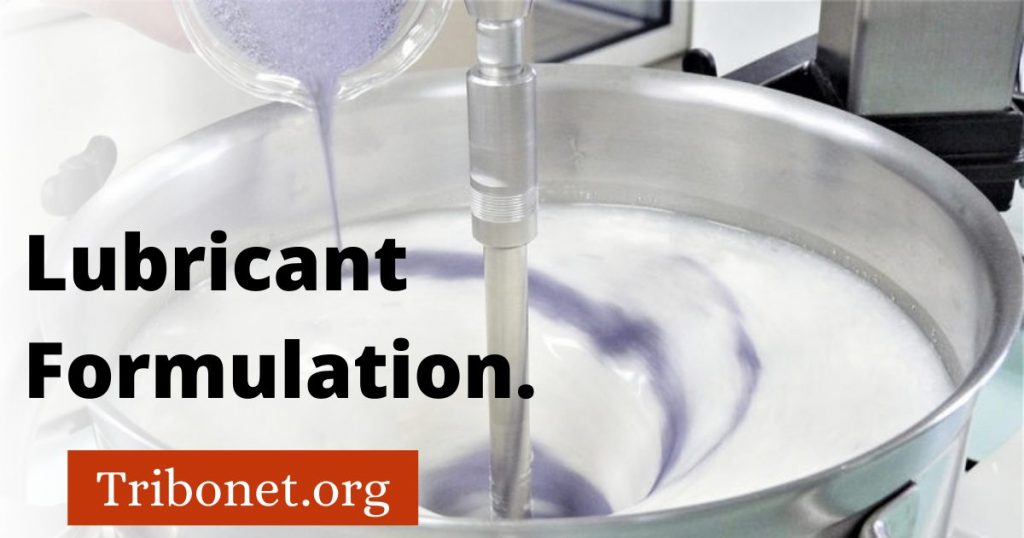The image depicts an industrial lubricant formulation process. Dominating the scene is a large silver mixing pot equipped with a mechanical stirring device at its center. Within the mixing pot, a white liquid is being vigorously mixed as violet-colored granules are poured into it, creating a swirling mixture of white and violet hues. Positioned towards the bottom left of the photo, there is text in bold black font that reads "Lubricant Formulation." Below this text is an orange rectangle containing the website "tribonet.org" written in white text. The overall setting suggests a high-tech lab environment, emphasizing the meticulous process of creating a specialized lubricant formulation.